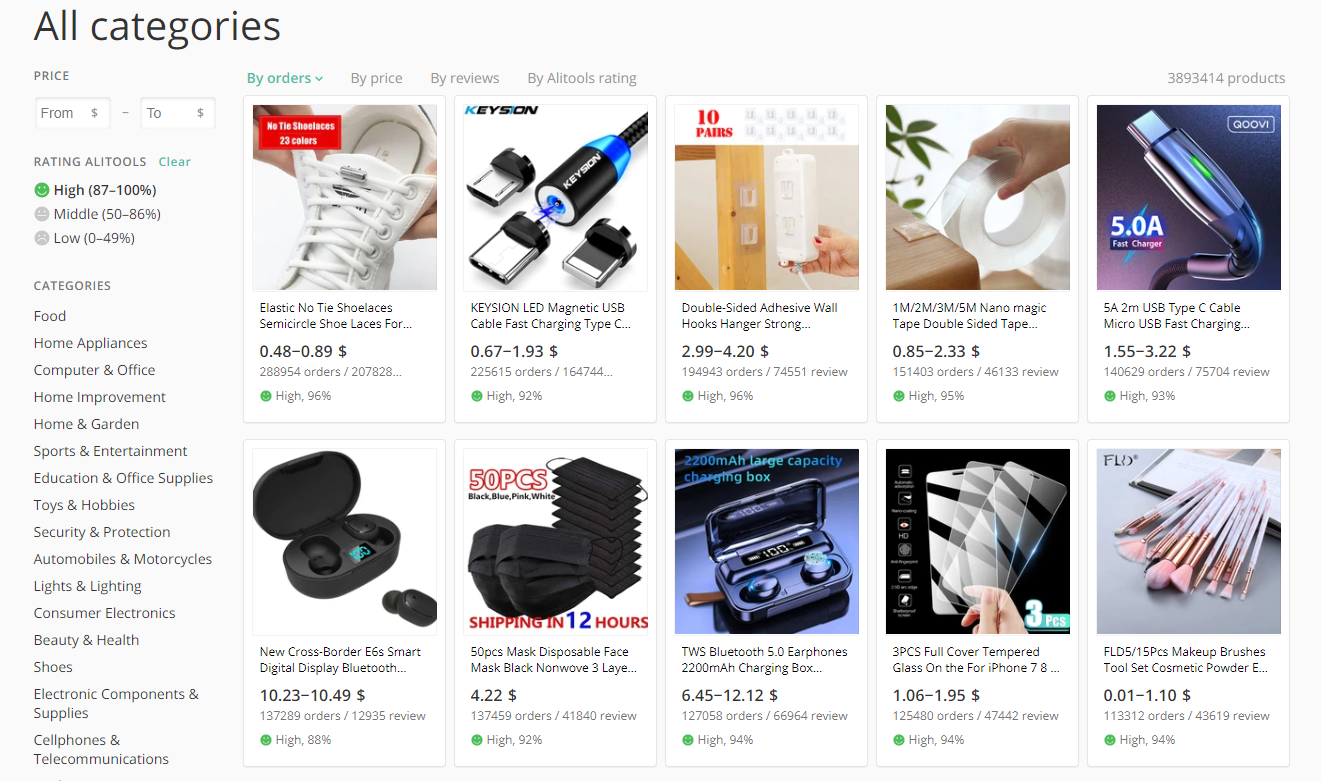Screenshot of an online shopping site displaying a variety of items. The page features a menu labeled "All Categories" at the top left, which has been selected to show a wide array of products. The background is white, adding clarity to the numerous items listed, each with their own thumbnail image and brief description. Notable products include white elastic no-tie shoelaces for sneakers, a fast-charging cable, double-sided adhesive wall hooks, magic double-sided tape, and USB-C charging cables. Among the other diverse items are makeup brushes, tempered glass phone screen covers, wireless in-ear headphones, and black disposable face masks in a 50-piece pack, described as nano weave masks suitable for COVID-19 protection. Each item, though somewhat small and challenging to read in detail, represents a snapshot of the extensive range available under the selected "All Categories" view.